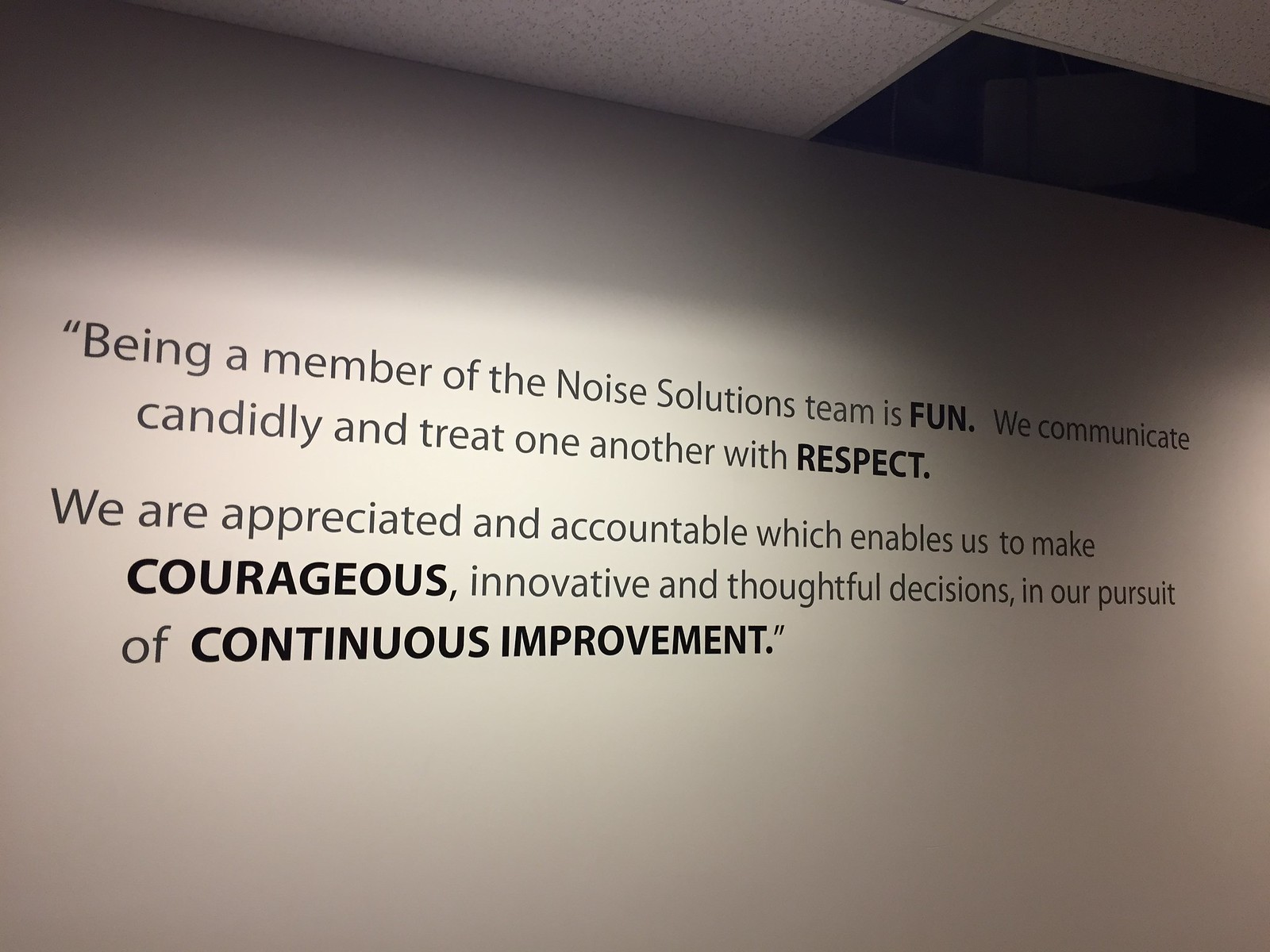The image portrays a section of a white wall featuring black text. The top part of the wall displays subtle shadows likely caused by overhead lighting. The ceiling is also partially visible in the frame. The wall is adorned with a quoted text that reads as follows:

"Being a member of the Noise Solutions team is fun" (with 'fun' in bold). "We communicate candidly and treat one another with respect" (with 'respect' in bold).

Following a space, the text continues on a new line:

"We are appreciated and accountable, which enables us to make courageous" (with 'courageous' in bold), "innovative, and thoughtful decisions in our pursuit of continuous improvement" (with 'continuous improvement' in bold).

The text concludes with an end quote. The bolded words emphasize key values and principles of the Noise Solutions team.